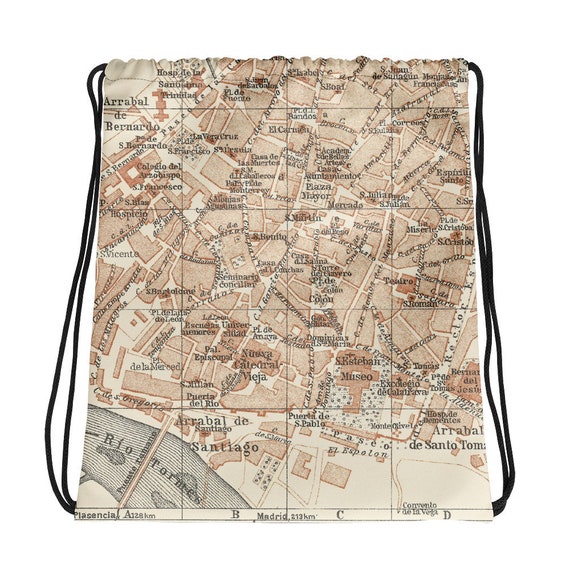The image depicts a detailed map with overlaid black grid lines, dividing the map into columns labeled A, B, C, and D along the bottom. The map's background is primarily light tan and dark tan shades, with building structures marked in salmon color. A significant feature of the map is a light blue river, labeled as "Rio Tornes," situated towards the bottom left, with a bridge crossing it. The map shows names of various places in black text, with one prominent name, "Santiago," visible in the B column near the river. Most of the map is densely populated with buildings, particularly towards the top, while the lower section appears more sparsely occupied. The image suggests that this map is printed on a drawstring bag, with evident black drawstrings on the sides and a gathered top, typical of such bags. The international nature of the map, along with the Spanish names, indicates it is likely not a U.S. locale. The image quality, however, is slightly blurry, making some of the smaller text hard to read.